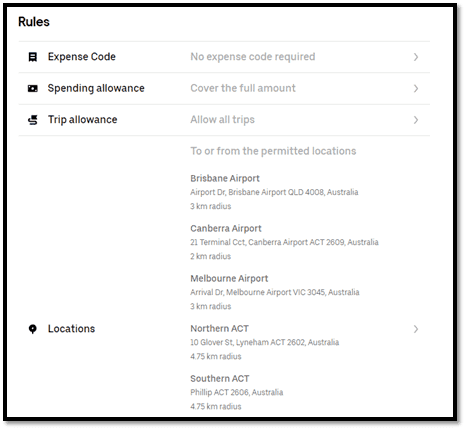This image is a detailed screenshot of a corporate business travel policy, outlining various rules related to expenses and allowances. The policy is divided into several distinct sections:

1. **Expense Code Requirement**: Indicates whether or not an expense code is necessary for a given transaction.
2. **Spending Allowance**: Specifies the amount covered by the spending allowance, stating that the full amount is covered.
3. **Trip Allowance**: Clearly states that all trips are allowed under this policy.
4. **Permitted Locations**: Lists specific addresses and defines permissible travel regions with a radius around several major Australian airports. The locations are detailed in an ascending to descending order, including Brisbane Airport, Canberra Airport, Melbourne Airport, Northern ACT, and Southern ACT.

The document appears to be part of a comprehensive travel management system, aimed at delineating where expenses are permitted and what allowances are available for business-related trips. The specific details and hierarchical organization suggest meticulous planning to facilitate seamless corporate travel and compliance with company guidelines.